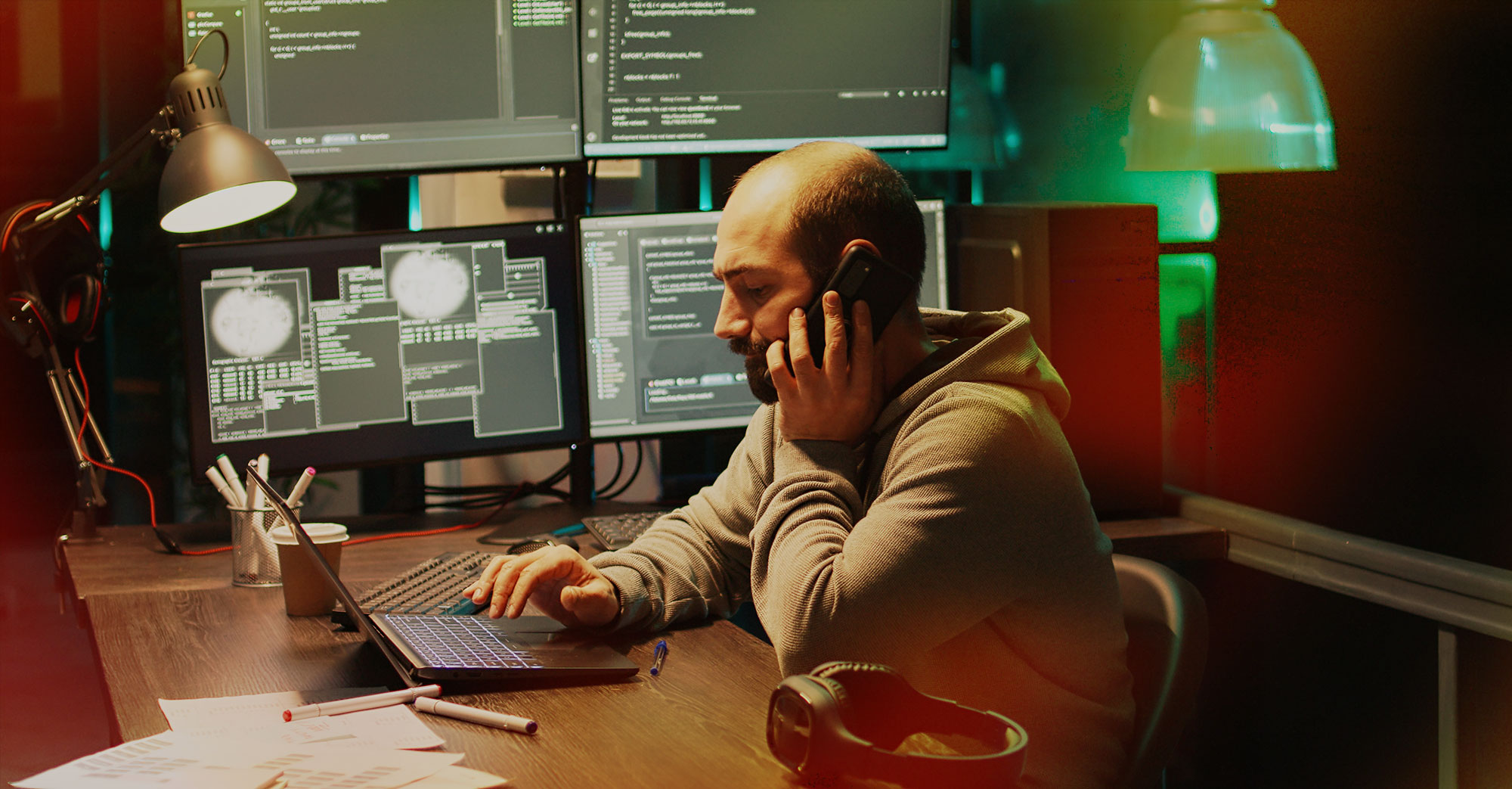In the image, a man with balding hair, a mustache, and a beard, is seated at a brown wooden desk in an office. He is wearing a gray hoodie and is engaged in a phone conversation on a black cell phone while simultaneously typing on a black laptop. The desk is well-equipped with various work materials: a clear silver cup holding multicolored markers, a cup of coffee, an array of pens and additional markers, and scattered papers, some of which appear crumpled. 

To his side, there are four computer monitors, arranged in two columns with two monitors each, all displaying different content. Two additional keyboards, presumably for the monitors, are also visible. A pair of headphones rests nearby. Overhead, a black dome light provides illumination, and in front of the man, a turned-on lamp further lights his workspace. The background features a mix of red and green lighting, adding a distinctive atmosphere to the office environment. Overall, the man appears focused and busy, multitasking between his phone call and his work on the laptop.